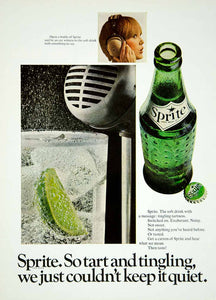This image is a vintage Sprite advertisement from a magazine, featuring a vertical rectangular layout with a light gray, almost off-white background. Occupying the top center is a small square photograph of a Caucasian woman facing right with short brown hair highlighted in front, and bangs. She wears over-the-ear headphones and gazes back over her shoulder. Below her image is a larger black-and-white rectangular photo of an old-fashioned silver microphone positioned above a clear glass filled with ice, a lime wedge, and a carbonated beverage resembling Sprite. To the right of this setup stands an iconic green Sprite bottle with a distinctly tall neck and textured bottom. The bottle is visibly opened, accompanied by a bent bottle cap on the ground beside it. The bottom of the advertisement features bold black text proclaiming the slogan: "Sprite, so tart and tingling we just couldn't keep it quiet."